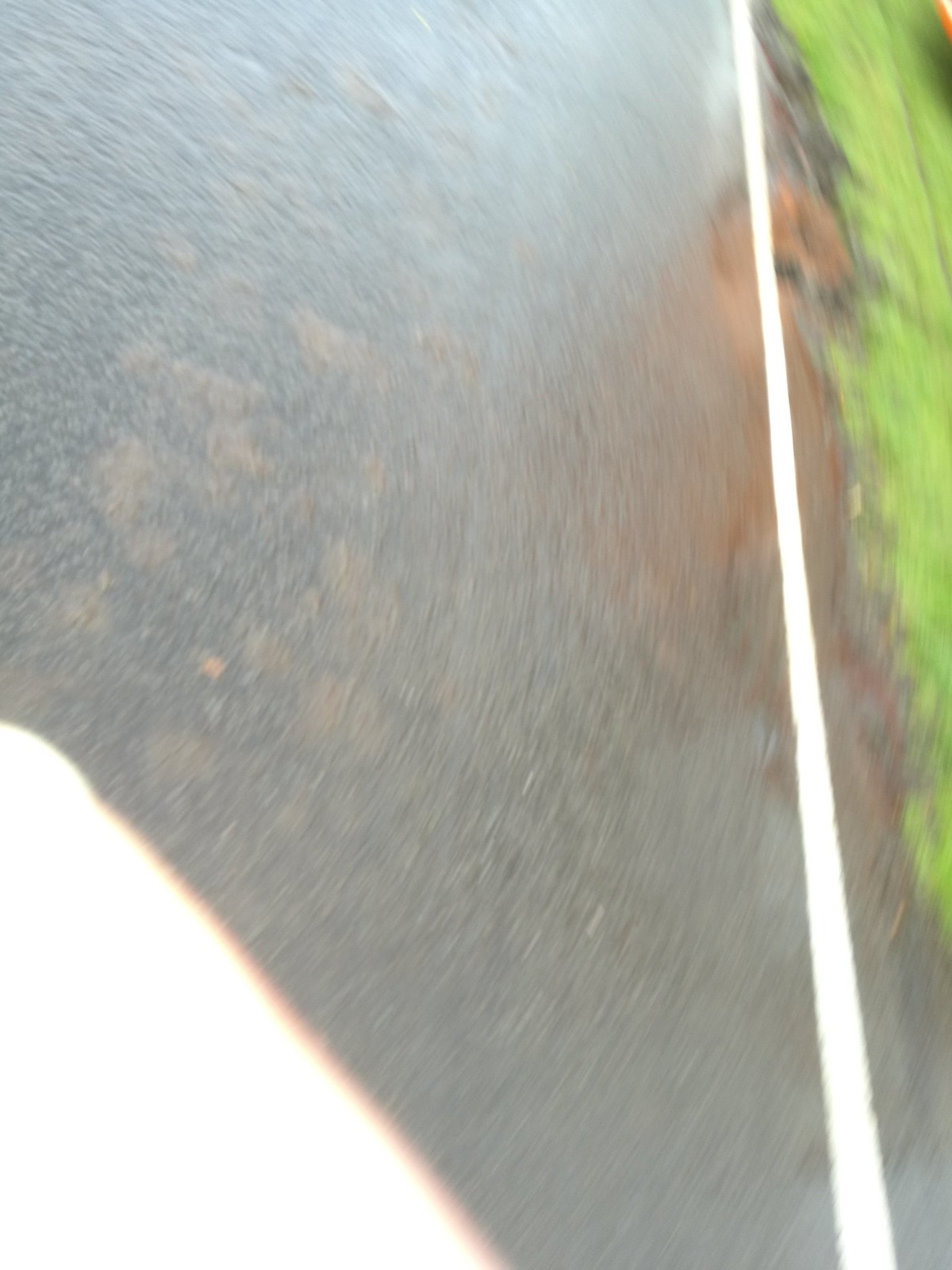In this blurry and low-quality photo, likely taken accidentally while moving or walking, we see a wet, grayish asphalt road with intermittent patches of brown interspersed. The pavement showcases a prominent white stripe, denoting a lane edge, which runs vertically up the right side of the image. Adjacent to this stripe, the tarmac displays lighter brown hues towards the middle before it transitions into a green, grassy verge. The right edge of the scene is dominated by this vivid green grass, interspersed with a slight grayish tinge at the transition point between the road and the lawn, possibly indicative of a suburban front yard. A segment of the lower-left corner of the photograph is obscured by a blurry white wedge, likely a finger or a part of the camera, contributing to the overall amateurish quality of the snapshot. Additionally, there is a reddish blur towards the upper right, which might be interpreted as an object or even an animal like a fox or dog, though the details are indiscernible due to the image's poor clarity.